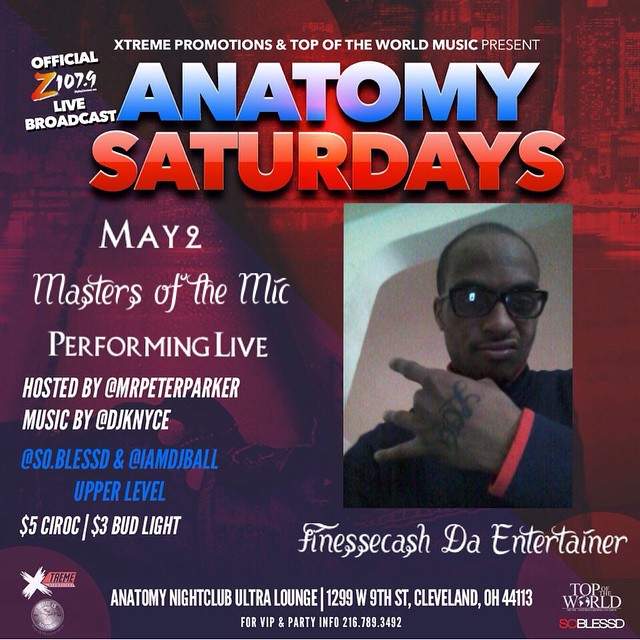This is a square advertisement poster featuring a vibrant background with shades of red, purple, and black, possibly depicting a skyline. At the top, white all-caps text reads "Extreme Promotions and Top of the World Music Present," followed by larger blue and white all-caps text announcing "Anatomy Saturdays." To the left of this, in white text, it states "Official Z107.9 Live Broadcast" with a distinctive yellowish-orangish "Z."

Below this, on the left side, the poster lists event details: "May 2nd," and "Masters of the Mic, performing live," hosted by "@MrPeterParker." Additionally, it mentions "Music by @DJKNYCE, @So.Blessed, and @IMDJBall," with "Upper Level" also noted in blue text. Promotional drink specials include "$5 Ciroc" and "$3 Bud Light."

The right side of the poster features a rectangular image of an African-American man with short hair and black-rimmed glasses, wearing a black top with red trim around the wrists. He is striking a hand gesture with his left hand, showing a tattoo on the top of his palm. Beneath his image, it reads "Finesse Cash, The Entertainer."

At the bottom of the poster, white text provides the venue details: "Anatomy Nightclub Ultra Lounge, 1299 West 9th Street, Cleveland, Ohio, 44113," with contact information for "VIP and Party Info: 216-789-3492." The bottom corners of the poster feature additional logos and text, with "Extreme" and "Top of the World" mentioned in white and red lettering.